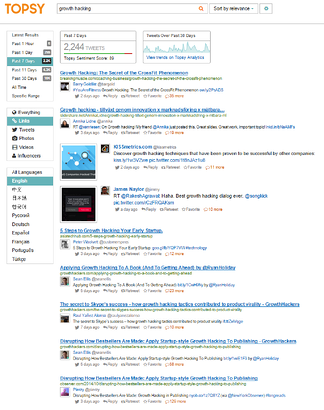The image clearly displays a detailed interface of an analytics dashboard focused on tracking the topic of "growth hacking" over the past seven days. On the right side, there are settings and a relevance drop-down box. On the left side, various time frames are presented, including "Past one hour," "Past one day," "Past seven days" (highlighted in blue), "Past 11 days," "Past 30 days," "All time," and "Specific range." The "Past seven days" view reveals a total of 2,300 mentions, displayed as "2.3K."

Below these time frames, there's another section that filters content into "Links," "Tweets," "Photos," "Videos," and "Influencers," with "Links" currently highlighted in blue. The interface is set to English, showing relevant search results for "growth hacking." A large box indicates that there have been 2,244 tweets about growth hacking in the past seven days, accompanied by a "Topsy Sentiment Score" of 89, and a line graph charting the trend of tweets over the last 30 days.

Underneath this data visualization, there are nine distinct articles related to growth hacking, each with a blue hyperlink for access, a snippet from the article, and information about the originating Twitter user. This section also offers options to reply, retweet, or favorite each article, facilitating engagement and further exploration.